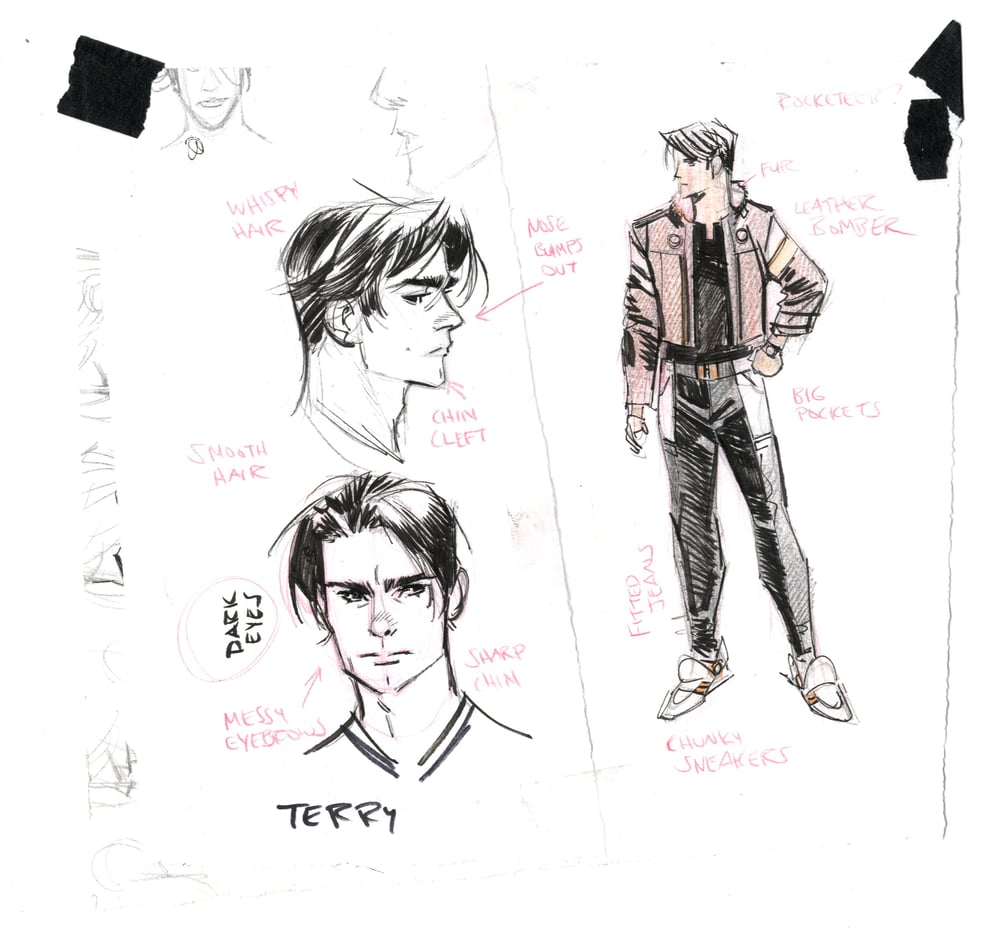This image showcases a detailed design sketch of a character named Terry. On the left side of the paper, there are two close-up drawings of Terry's face and upper chest, featuring annotations in red and black ink. The top sketch highlights Terry's smooth hair, a cleft chin, wispy hair, and a nose that bumps out, indicated by red arrows. Below that, a frontal view of Terry's face includes notes on his messy eyebrow, sharp chin, and dark eyes. The name "Terry" is inscribed at the bottom in bold black lettering. Additional faint sketches and a shaded black square occupy the top left corner.

On the right side of the paper, a full-body drawing displays Terry in a completed and colored form. He is outfitted in a tan jacket with white and yellow stripes, a black shirt, black fitted jeans with visible white pockets, a gray belt, and white, slightly pointed sneakers. Red annotations label various details such as "big pockets," "leather bomber," "fur," and "chunky sneakers." This thorough depiction of Terry, drawn on a white background, provides a comprehensive view of the character’s design, capturing both close-up and full-body perspectives.